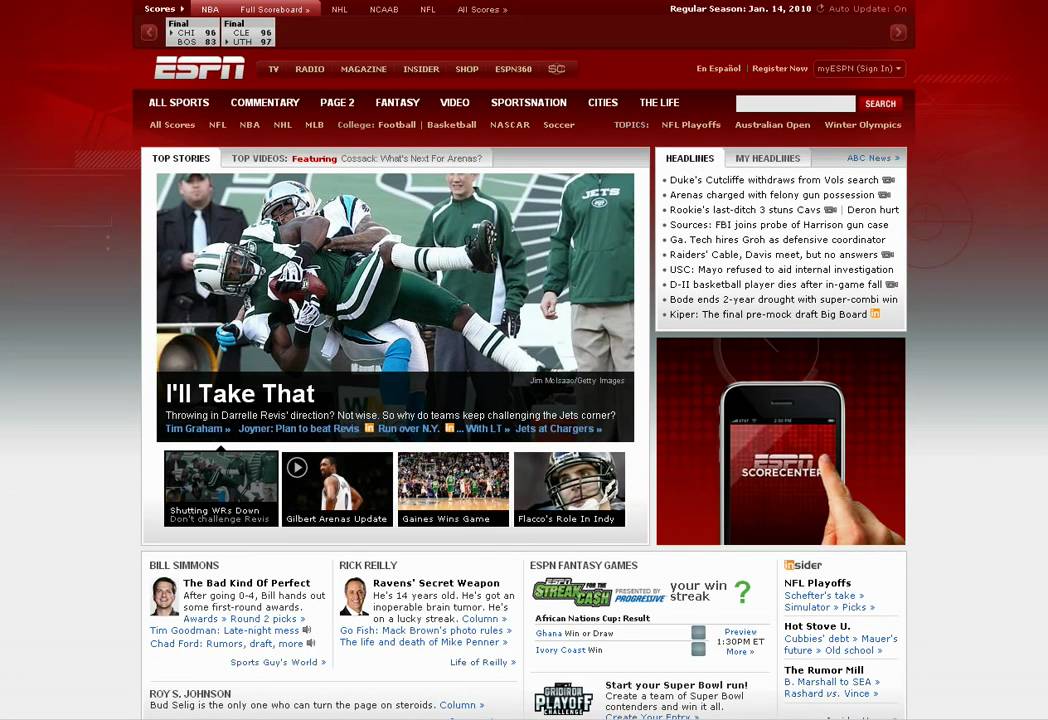This post features a screenshot of what appears to be an outdated ESPN webpage, identifiable by its dated advertisements and design reminiscent of early 2010s web layouts. ESPN, primarily a sports news channel focusing on American sporting events, showcases a main news article featuring a high-resolution photo from a football game. The image highlights a team in green uniforms, likely the New York Jets, competing against another team whose identity is unclear but could possibly be the Detroit Lions, suggested by a player wearing a light blue uniform. In addition to the main story, the webpage also includes smaller sections displaying various sports events and news from around the country, reflecting the diverse range of coverage provided by ESPN.